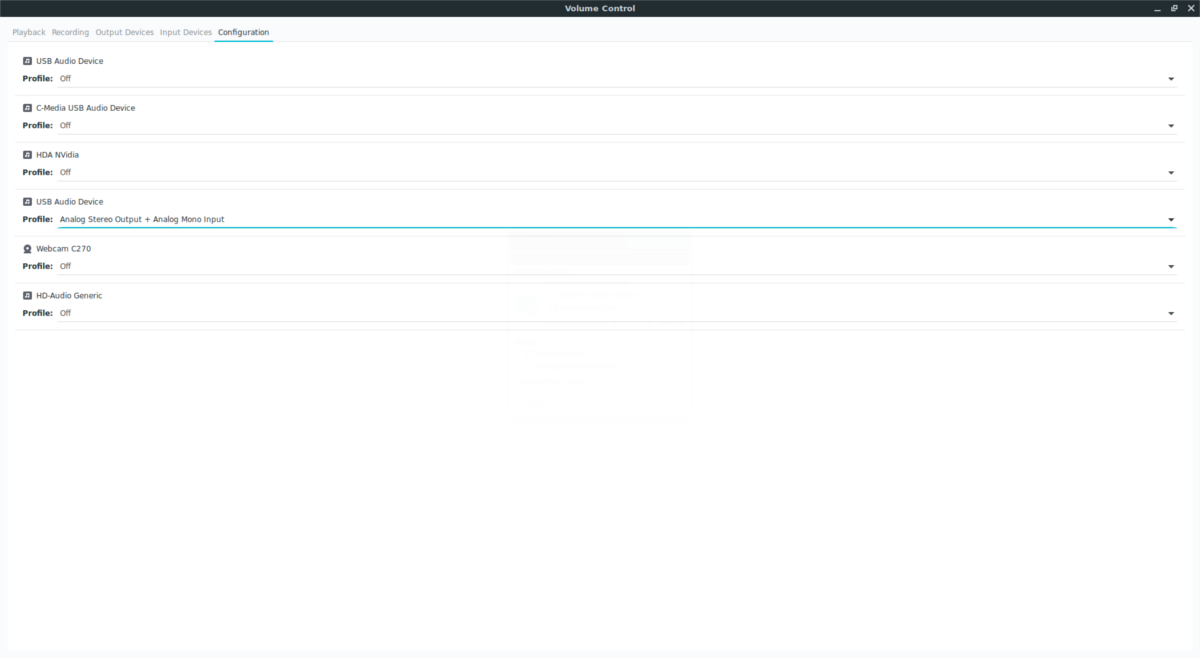The image showcases a settings interface for an audio program or editing tool. At the top, a black bar labeled "Volume Control" features a small 'X' icon. Below this header, there are several options related to audio device settings, with extremely small and hard-to-read text.

The first option available is to "Use Audio Device," which offers various audio profiles. Each profile has a downward-facing arrow, allowing users to access a dropdown menu for selecting their preferred setting. The profiles listed include:

1. **HCA Audio** - The user can click to choose from options such as "Analog." A blue line highlights this section indicating it's the active selection area.
2. **USA Audio Device** - Similar to the HCA Audio, this profile also has a downward arrow for selecting different audio preferences.
3. **HQ Audio** - Labeled as "Generic," this section allows users to choose their desired audio settings via another dropdown menu.

Additionally, there is a mention of a "Webcam" setting, though the numbers next to it are illegible. Like the audio settings, this also provides a dropdown menu for selection.

The entire interface is presented on a white background with no shading, adding to the difficulty of reading the small text.